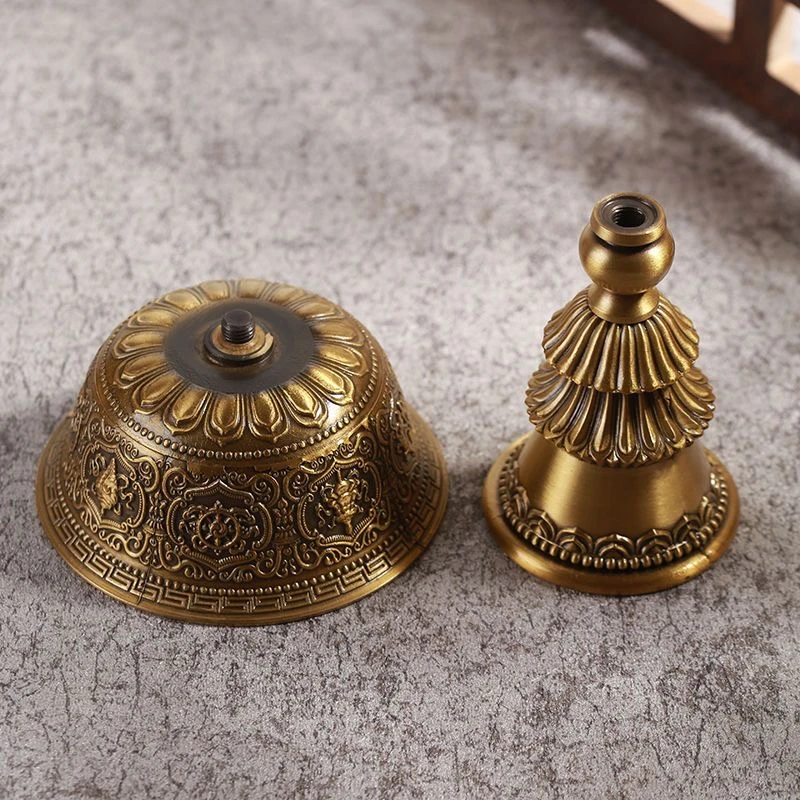The photograph depicts an intricately detailed, antique-looking object disassembled into two parts, resting on a mottled grey and white marble surface. The larger piece, on the right, has a tall, triangular base with two layers resembling upside-down flowers and flares out at the bottom like a bell. Made of bronze, this base is adorned with elaborate carvings, including a bunch of grapes and a shield. The second piece, on the left, is similar to an upside-down bowl and appears to be the top part, with a small black bolt protruding from its center. This piece also features intricate engravings and is believed to fit into the base, akin to a fancy, antique door knob or perhaps the handle of a ceremonial bell.